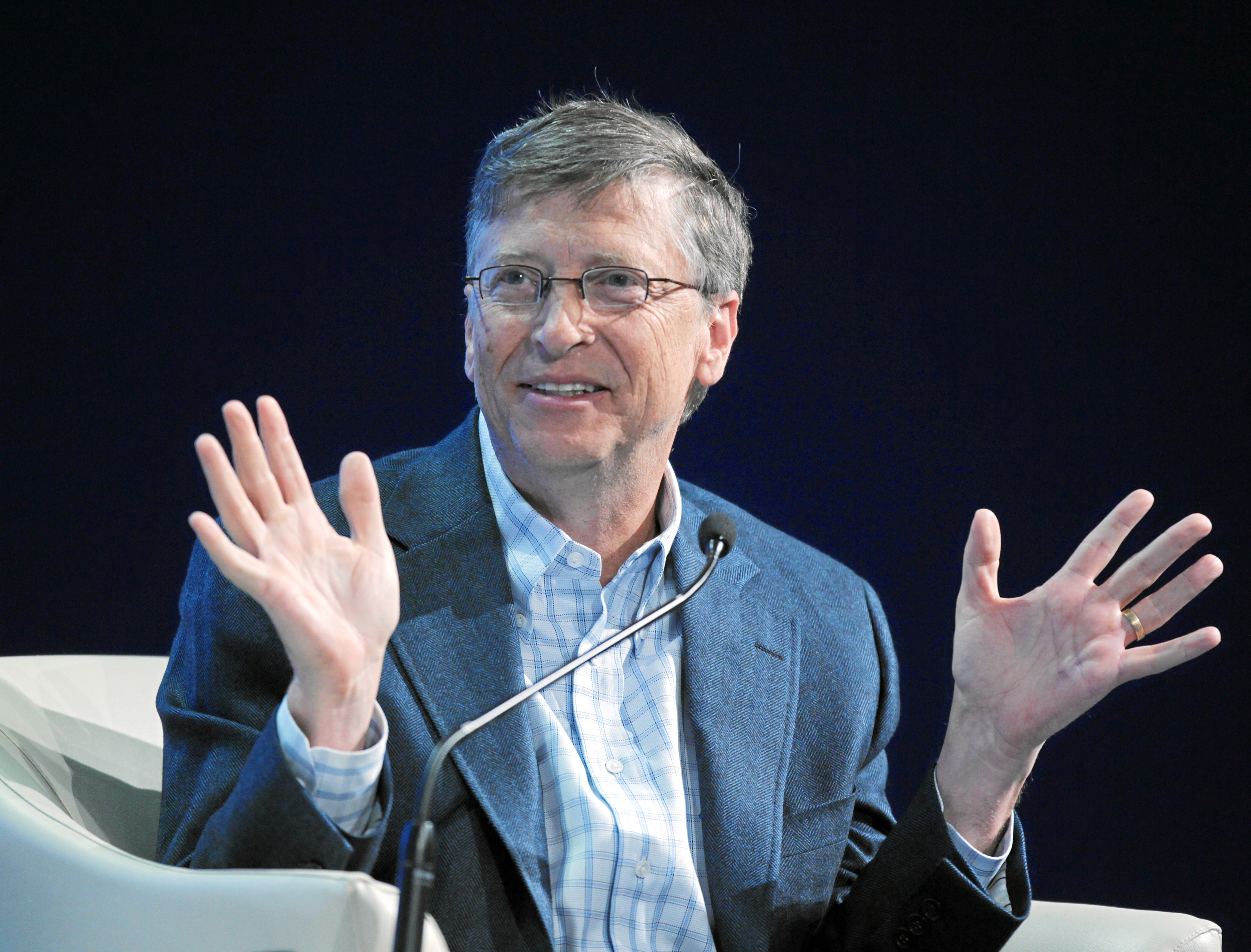The image captures Bill Gates, the Microsoft founder, seated in a white chair, with a comfortable, rounded back. His gray hair and black wire-frame glasses stand out as he smiles warmly, exuding confidence. Sporting a blue suit jacket over a checkered white and light blue dress shirt with the top button undone, he appears both relaxed and presentable, lacking a tie. Gates' expressive demeanor is evident as he raises both hands, elbows bent at his sides, with palms open. A gold wedding ring adorns his left hand. To his side, a black microphone hints at a stage setting, potentially for a presentation or debate. The surroundings include a backdrop of deep blue curtains, accentuated by focused lighting that illuminates Gates, adding to the formal yet inviting atmosphere.